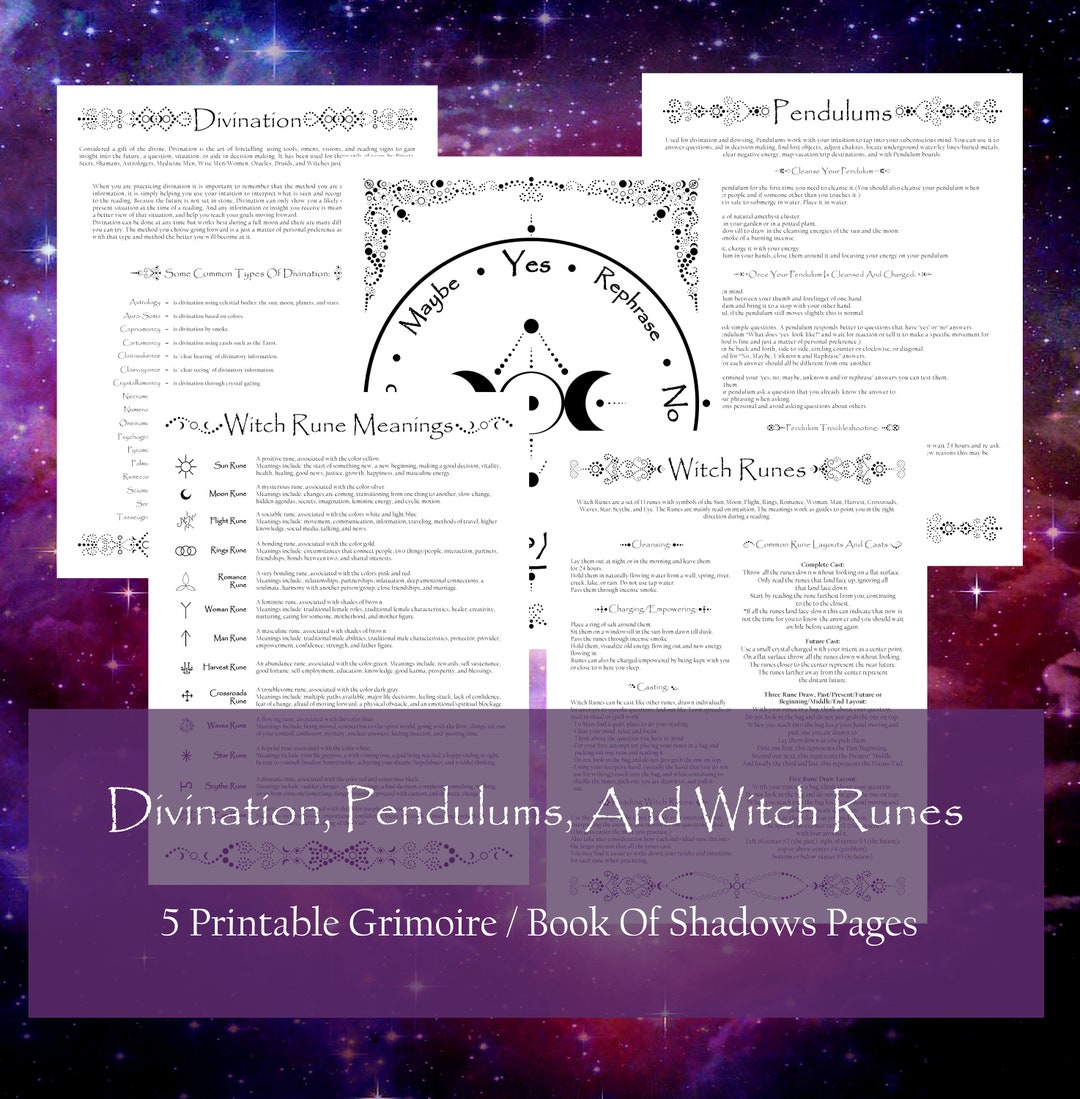The image depicts an advertisement set against a starry, galaxy-themed background with hues of purple, blue, and black. The backdrop is sprinkled with numerous stars, enhancing the mystical ambiance. In the foreground, there are five white cardboard cards arranged in a slightly overlapping manner, presenting various topics related to witchcraft and divination. The cards are labeled as follows: "Divination," "Pendulums," "Witch Rune Meanings," "Witch Runes," and a final card in the center which displays a black and white circular diagram with the words "maybe," "yes," "rephrase," and "no" along its edge. At the bottom of the image, a transparent purple bar holds a white text caption stating, "Divination, Pendulums, and Witch Runes. Five Printable Grimoire/Book of Shadows Pages." Together, these elements showcase five printable pages designed to offer detailed information on various divination practices, specifically focusing on witchcraft runes, pendulums, and spells.